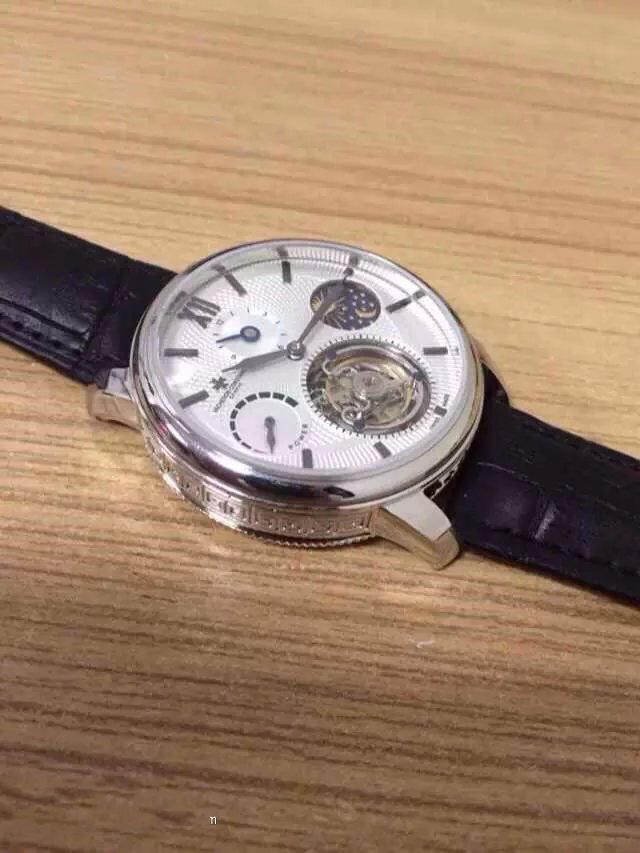A light brown table counter with distinctive striped etchings forms the background of this image. At the center of the counter lays a watch, prominently displayed with its black band fully extended; the band stretches out to the left and right sides of the image. The circular watch face is encircled by a silver bezel adorned with fine etchings, giving it a refined look. The face of the watch features four smaller sub-dials, adding complexity to its design. The hands of the clock, also in silver, stand out against the face, making the time easily readable. The overall composition highlights the intricate details of the watch against the textured surface of the counter.